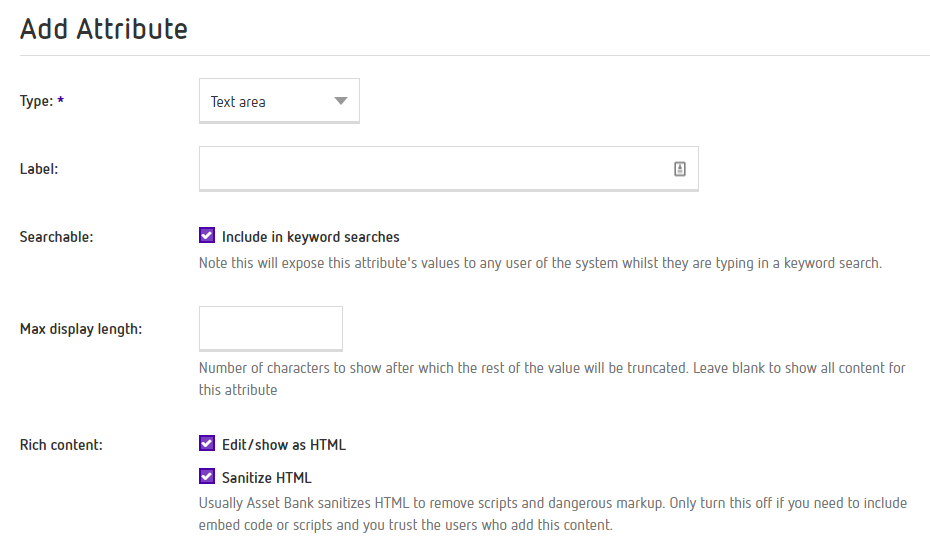The image displays a user interface for adding an attribute, positioned in the upper-left corner of a white background, where the largest and prominent text reads “Add Attribute” in black font. Below this, a gray line divides the section, followed by a left-justified layout. The first element is a dropdown menu labeled "Text Area" in a smaller font. The label is followed by a data field on the left, adjacent to an unclear element on the right.

Next, the interface shows an option labeled "Searchable" with a checked box that reads, "Include in keyword searches." An accompanying note explains that this option will expose attribute values to any system user conducting a keyword search.

Further down, a field labeled "Max Display Length" is present, offering a data input area for specifying the number of characters to display before truncation. The note clarifies that leaving this field blank will display all content for the attribute, and currently it is left blank.

The section titled "Rich Content" provides settings for content formatting. It has options like "Show Editor" and "Edit/Show as HTML," both of which are ticked, along with "Sanitize HTML." A description explains that sanitizing HTML removes scripts and dangerous markup, advising to turn this off only if you need to include embedded code or scripts and trust the content contributors.

The color scheme of the interface is predominantly black, white, gray, and purple.